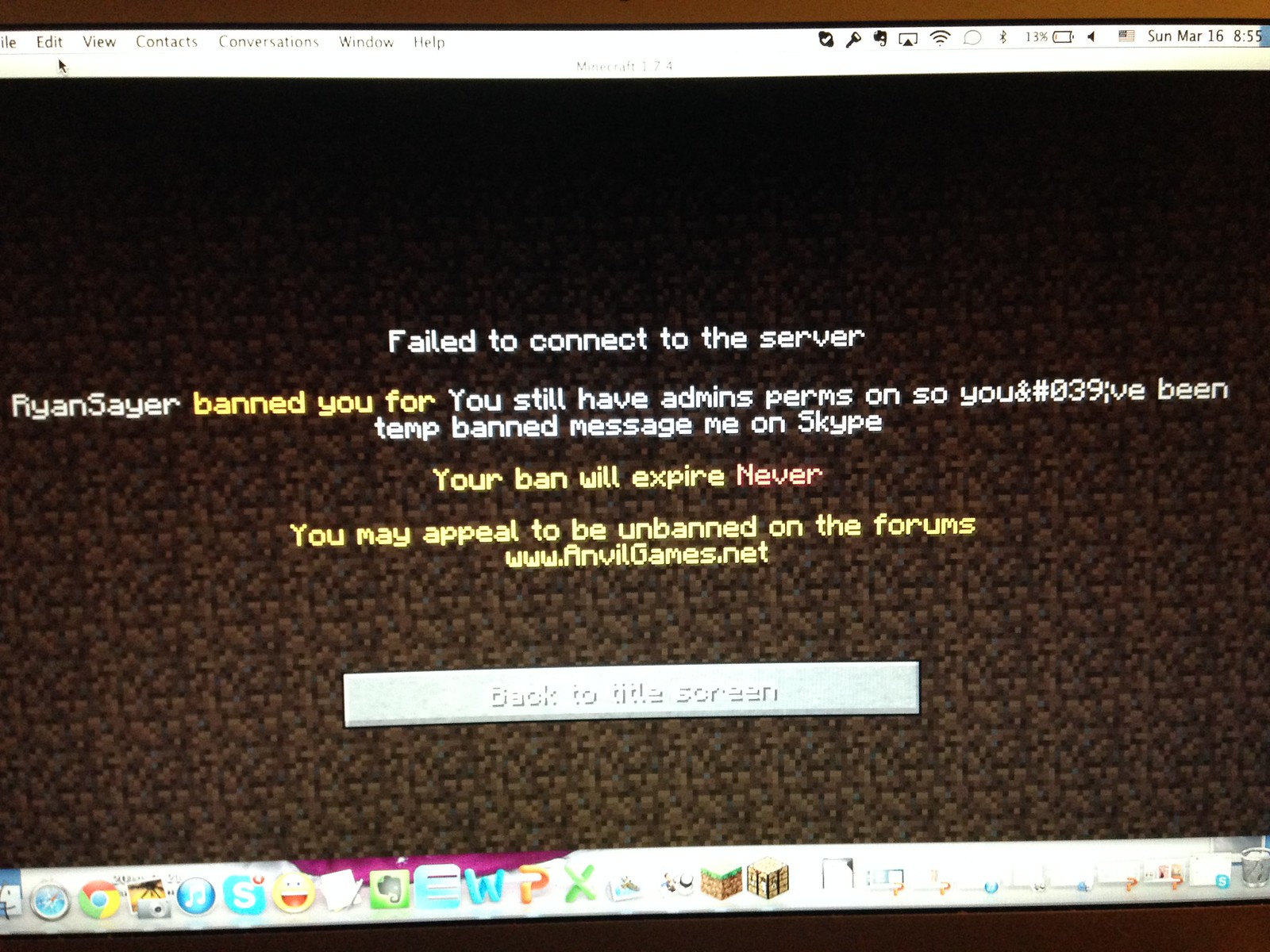The image is a screenshot of a computer desktop displaying an error message from what appears to be Minecraft, as indicated by the 64-bit dirt wall background, resembling a brown carpet. The screen prominently features white text in a DOS-like font that reads: "Failed to connect to the server. Ryan Sayer banned you for you still have admin's perms on so you and Lumber039 have been temp banned. Message me on Skype. Your ban will expire later. You may appeal to be unbanned on the forums www.finwheelgames.net." At the bottom of the screen, below the error message, is a long white button labeled "Back to the Title Screen." The image is framed by the Windows taskbar, which is also displayed in white.